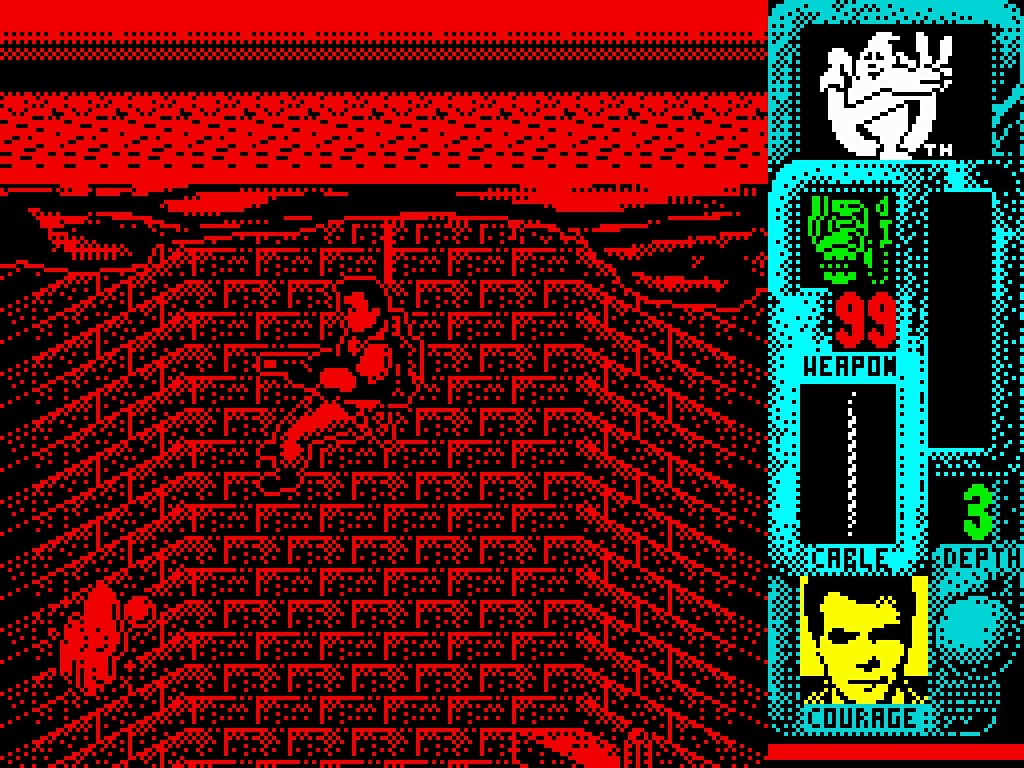An in-game screenshot from a nostalgic Sega Mega Drive title, likely a Ghostbusters game, makes for a visually intense scene. Dominating the view, red and black pixels create a wall-like structure that spans three-quarters of the screen, showcasing a complex pattern of dots and dashes. Hovering midway up this wall, a character equipped with a jetpack and a gun, presumably a Ghostbuster wielding ectoplasm equipment, prepares for action. In the lower-left corner, an eerie ghost with a bizarre, smiling face menaces the scene. The right side features the iconic Ghostbusters logo, unmistakably confirming the theme. The game graphics, typical of 1990s 16-bit era design, evoke a sense of thrilling, pixelated nostalgia.